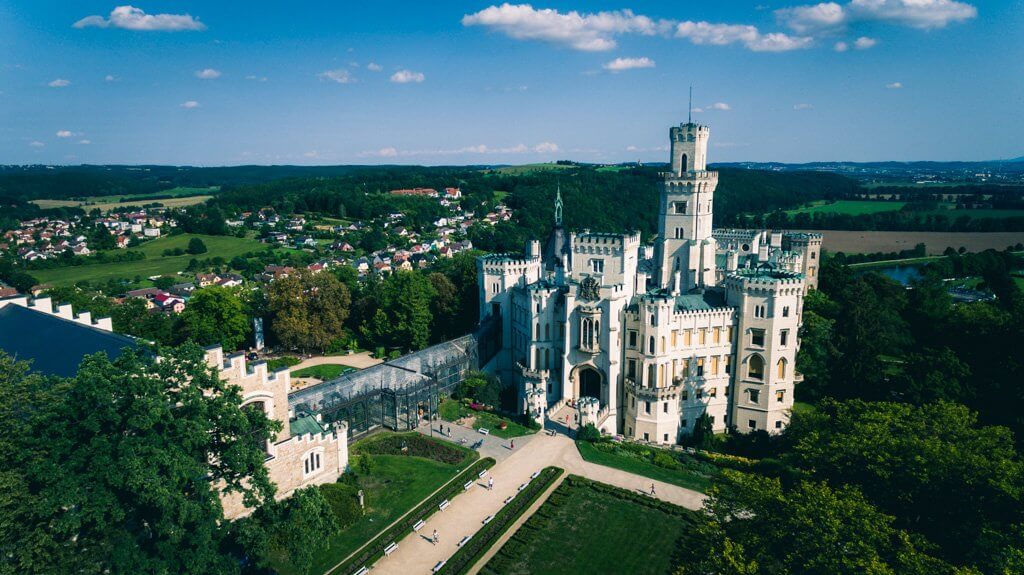The photograph showcases a grand, old white castle set in a lush valley, surrounded by abundant greenery. The castle, an expansive multi-story structure, features yellow window trim and a high central tower. To the left of the castle, there is another building with yellow brick and white trim, and what appears to be a gate. Various walkways converge at the castle, where several people can be seen strolling. The left side of the image also reveals a village with numerous white-and-red-roofed structures, while the right side is dominated by trees. The horizon boasts a clear blue sky adorned with fluffy white clouds. In front of the castle, neatly manicured green lawns and gray sidewalks guide visitors around the area, leading to additional green fields and a possible farming area in the distance.